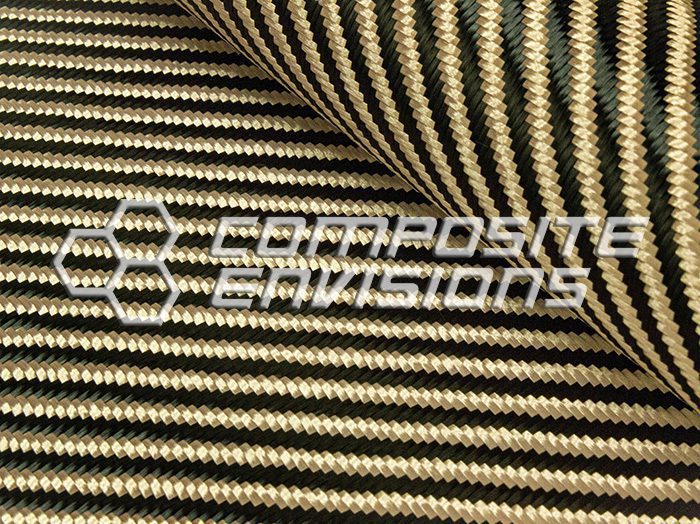The image features a central, slightly transparent watermark text that reads "Composite Envisions" in capital letters with a dark gray, somewhat 3D appearance. To the left of the text are three small, connected hexagons resembling a honeycomb, in the same color as the text. The background appears to be a shiny, composite material that is black with various shades of brown—specifically, dark brown, light brown, and tan. This composite material has a layered, book-page-like effect, as if peeling back a top layer to reveal an identical patterned layer beneath. The overall aesthetic might be digital, potentially created with computer graphics, and evokes the texture of a textile or woven fabric.